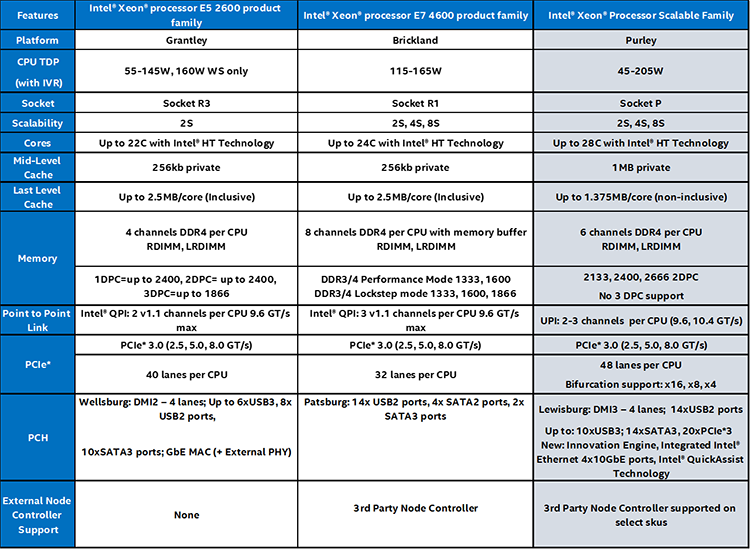The image is a detailed product comparison chart capturing various specifications and features of three different Intel Xeon processor families. The chart, seemingly sourced from a computer or website, features four vertical columns. The far-left column, set against a blue background with white text and black borders around each rectangular section, lists categories such as Features, Platform, CPU, TDP (Thermal Design Power), Socket, Scalability, Cores, Mid-Level Cache, Last-Level Cache, Memory, Point-to-Point Link, PCIe, PCH, External Node, and Controller Support. 

At the top of the next three columns, the chart titles each corresponding section with the product names: Intel Xeon Processor E5-2600 Product Family, Intel Xeon Processor E7-4600 Product Family, and Intel Xeon Processor Scalable Family. These columns provide a detailed comparison of the specified features and specifications for each product. The E5-2600 series uses the Grantly platform, the E7-4600 series utilizes the Brickland platform, and the Scalable Family operates on the Purley platform. 

Further details in the chart indicate differences in memory channels — the E5-2600 features four channels, the E7-4600 supports eight channels, and the Scalable Family has six channels. Other shared metrics include cache sizes, CPU capabilities, and scalability options, assisting users in determining which processor family best meets their specific requirements.